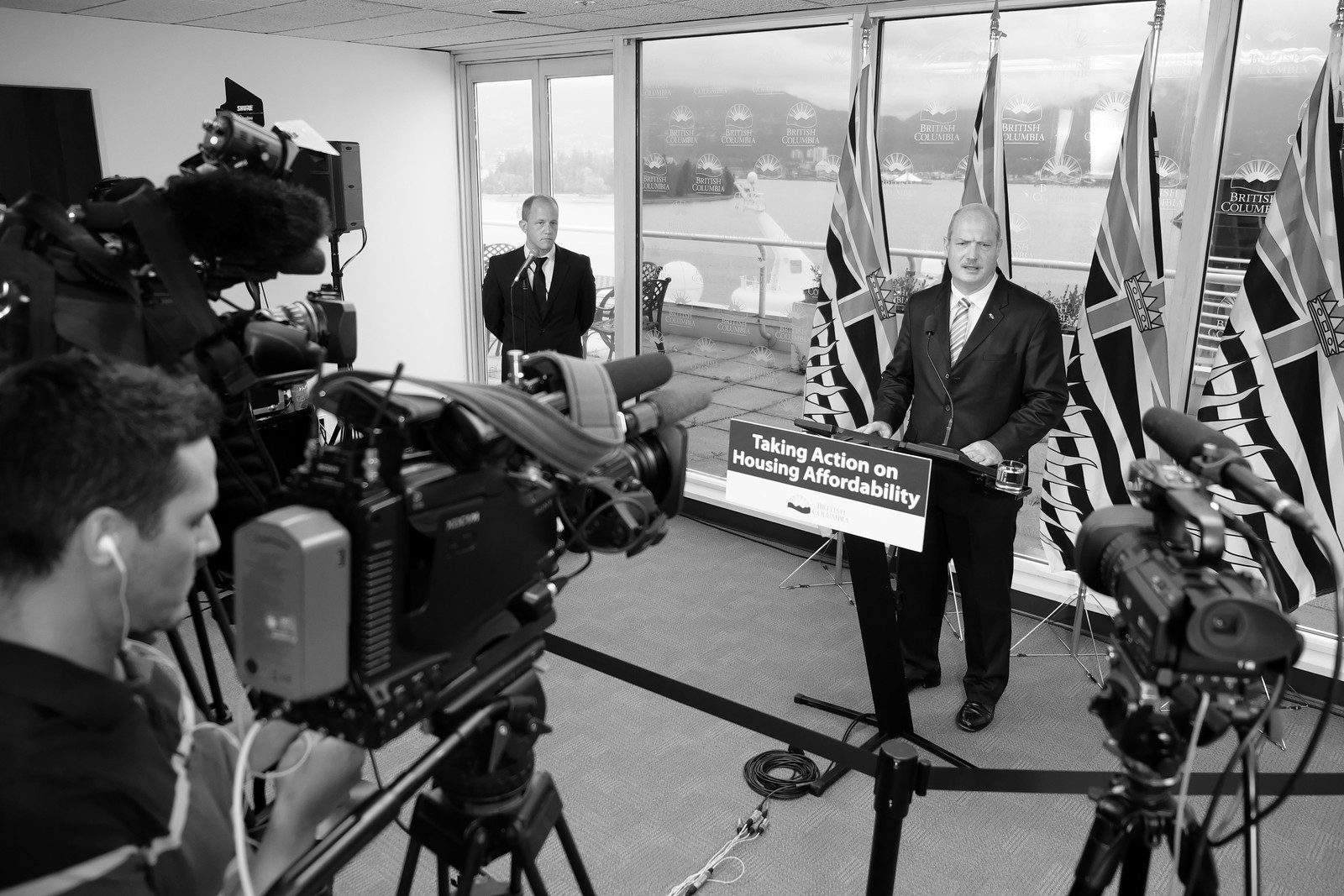The black-and-white photograph captures a news interview set in a room with large windows that open up to an ocean bay, with a few boats visible in the distance. A balding gentleman in a black tuxedo stands at a podium, which displays a sign reading "Taking Action on Housing Affordability" in white font on a black background. Behind him are four British flags. In front of him, there are three cameras, and an individual is actively filming the scene. On the left side of the image, another man in a black tuxedo stands watching. Additionally, a black fence is set up around the border where the speaker is standing. The setting suggests a formal event focused on housing issues, with a significant amount of media coverage.